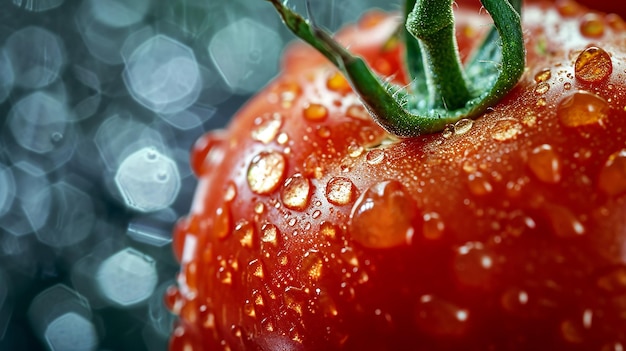This professionally taken close-up image of a tomato captures vivid details ideally suited for a casual restaurant like Fazoli's. The tomato, appearing massive due to the zoomed-in perspective, showcases the vibrant red skin adorned with numerous water droplets, both large and small. The green stem, with its four to five distinct segments, stands out, accentuating the freshness of the tomato. The droplets on the tomato's surface are sharp and clear, resembling a freshly rain-kissed look, while the subtle 'hairs' on the stem add an extra layer of detail. Background elements are blurred into dark tones with scattered white circles, mimicking the effect of sparkling glares or diamond-like sequins, emphasizing the tomato as the primary subject and giving the impression of rain. The meticulous focus on the central droplets and the stem, against a seemingly deeper blurry background, draws attention to the moist, juicy allure of the tomato, making it an eye-catching and appetizing image.